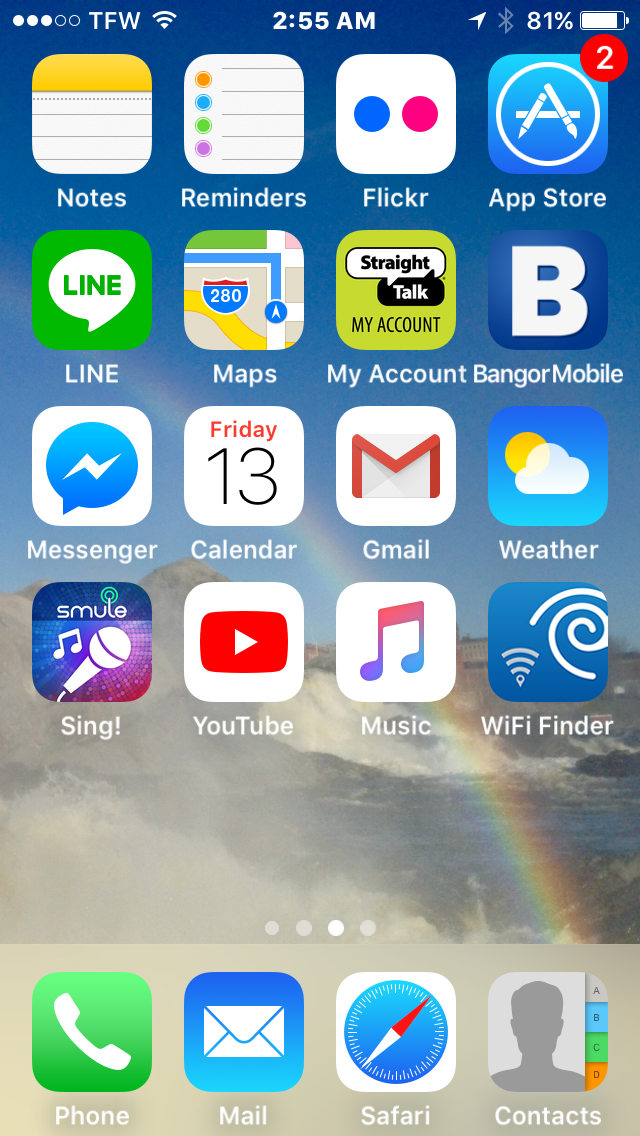The image is a screenshot captured from an iPhone, featuring a vibrant beach-themed wallpaper in the background. The wallpaper showcases majestic waves crashing against a rugged jetty, with a small rainbow emerging through the mist. Superimposed on this scenic backdrop are a total of 16 neatly arranged app icons, displayed in four rows and four columns. 

Starting from the top left corner and moving right, the first row features:
1. Notes - represented by a small notepad icon.
2. Reminders - another notepad with dotted lines.
3. Flickr - a white square with a distinctive blue and pink dot.
4. App Store - a familiar blue icon.

The second row includes:
5. Line - likely depicted by its green speech bubble.
6. Maps - the customary map representation.
7. My Account - an icon indicative of personal account management.
8. Banger Mobile - potentially a custom or lesser-known app.

The third row showcases:
9. Messenger - the recognizable speech bubble, likely blue.
10. Calendar - a grid or numerical date icon.
11. Gmail - typically a red envelope.
12. Weather - an image indicative of weather conditions.

The fourth and final row displays:
13. Sing - an app possibly related to music or karaoke.
14. YouTube - the iconic play button on red.
15. Music - likely represented by a musical note.
16. Wi-Fi Finder - an icon suggestive of Wi-Fi signals.

At the bottom end of the screen are the primary apps docked for easy access:
- Phone - the green handset icon.
- Mail - an envelope symbol.
- Safari - the compass icon.
- Contacts - a silhouette icon typically in a gray or blue background.

This detailed arrangement and selection of apps offer insight into the user's preferences and frequently used services, seamlessly integrated over the picturesque beach wallpaper.